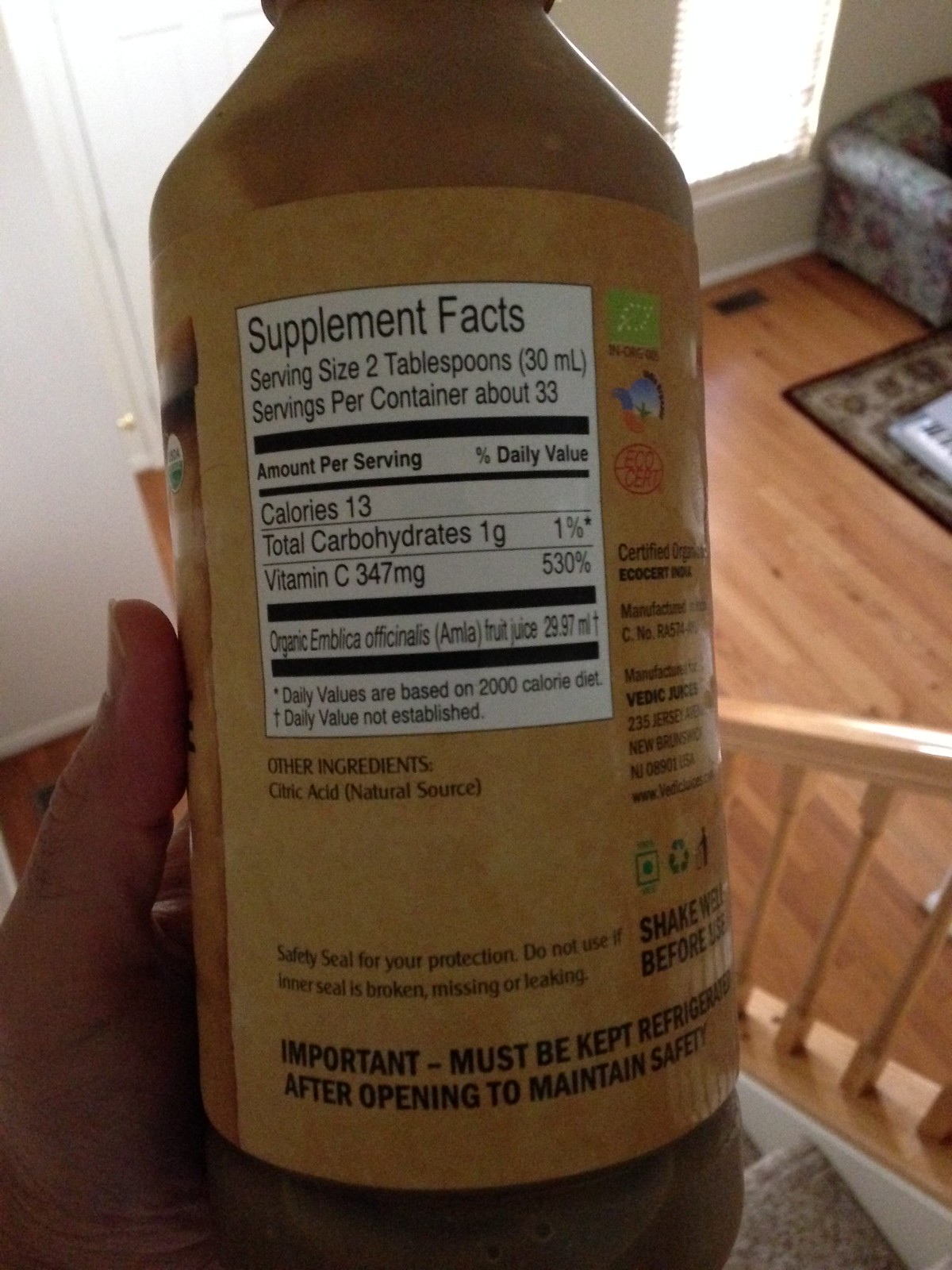In this image, a person is holding up a brown bottle with a white label that prominently displays Supplement Facts. The label details servings per container (about 33), serving size (two tablespoons), 13 calories per serving, one gram of total carbohydrates, and lists ingredients such as citric acid and vitamin C. The individual holding the bottle is using their left hand, suggesting a casual, personal setting, likely photographed with a cell phone camera. 

The background reveals the interior of a bright and sunny house or apartment. The setting features a wooden floor and a gray-carpeted staircase with a light brown, wooden banister. On the first floor, a window allows ample sunlight to illuminate the space, highlighting the arm of a sofa, a visible heating vent on the floor, and a section of a carpet. The detailed and cozy interior suggests a lived-in, comfortable home environment.